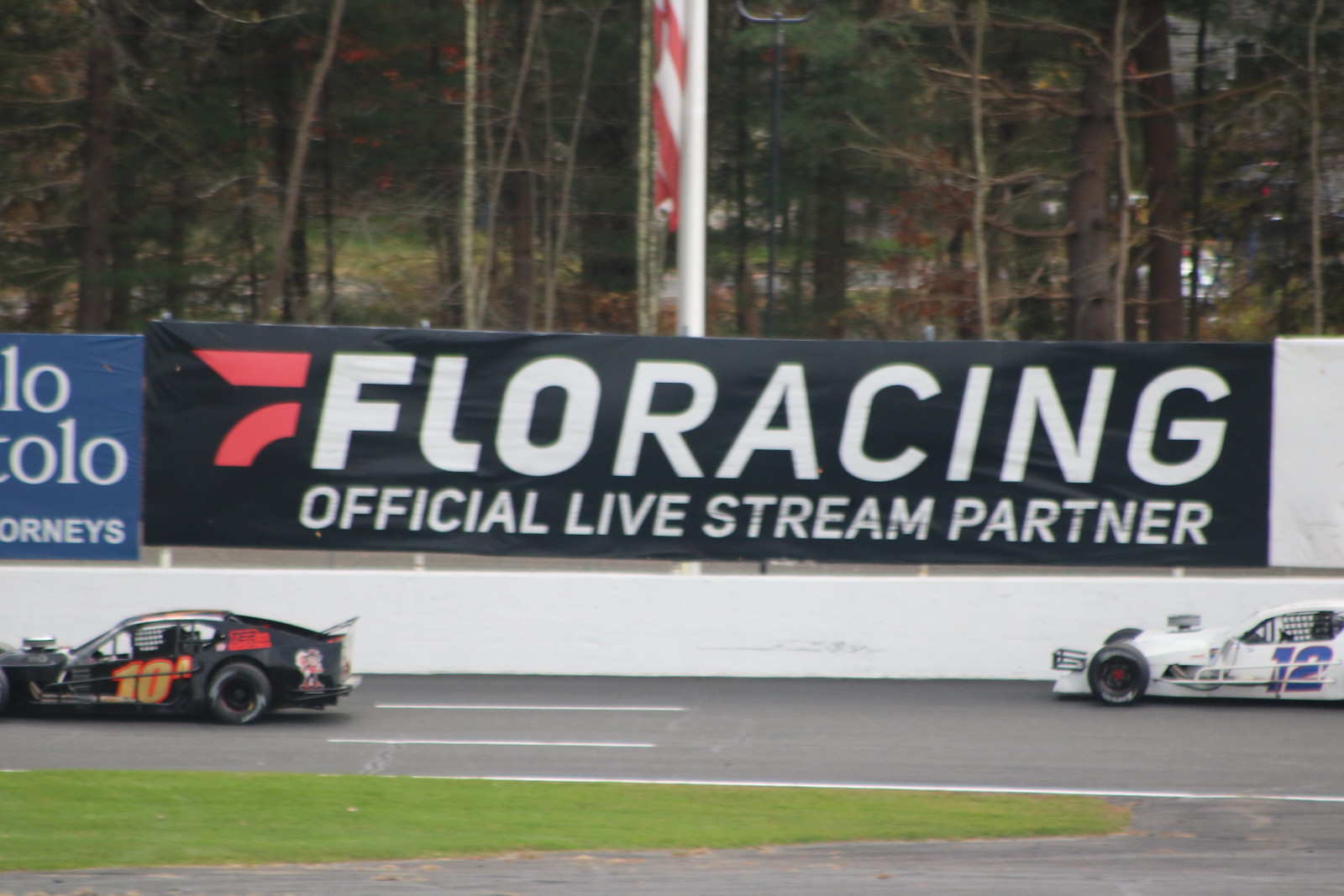This image captures an exhilarating moment on a racetrack, featuring two stock cars in the heat of competition. On the left, a black car with gold number "10" outlined in red surges forward, while on the right a white car bearing a blue number "12" follows closely behind. The race unfolds on a multi-lane asphalt track, with crisp white stripes marking the lanes. In the foreground, a patch of green grass contrasts with the gray asphalt. A towering white safety wall runs parallel to the track, and above it, a prominent black banner declares "Flow Racing, Official Livestream Partner" in bold white letters, accented with a small red design. The scene is set outdoors under daylight, and in the background, a dense cluster of trees provides a natural backdrop, adding green hues to the diverse color palette that includes shades of gray, white, black, gold, red, blue, yellow, and orange. Flags and other trackside objects are faintly visible in the distance, adding to the vibrant, bustling atmosphere of the race.